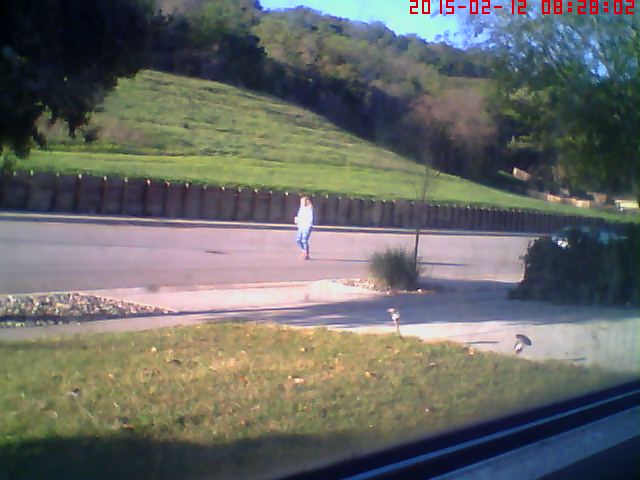A photograph captures a solitary figure walking down a city street, viewed through a window, which is partially visible at the bottom of the image along with a subtle reflection on the glass. The opposite side of the street features a wooden fence-like retaining wall, behind which a grassy hill ascends, dotted with lush green trees at the crest. A timestamp in red is embedded in the bottom corner, marking the moment as February 12, 2015, at 08:28:02.